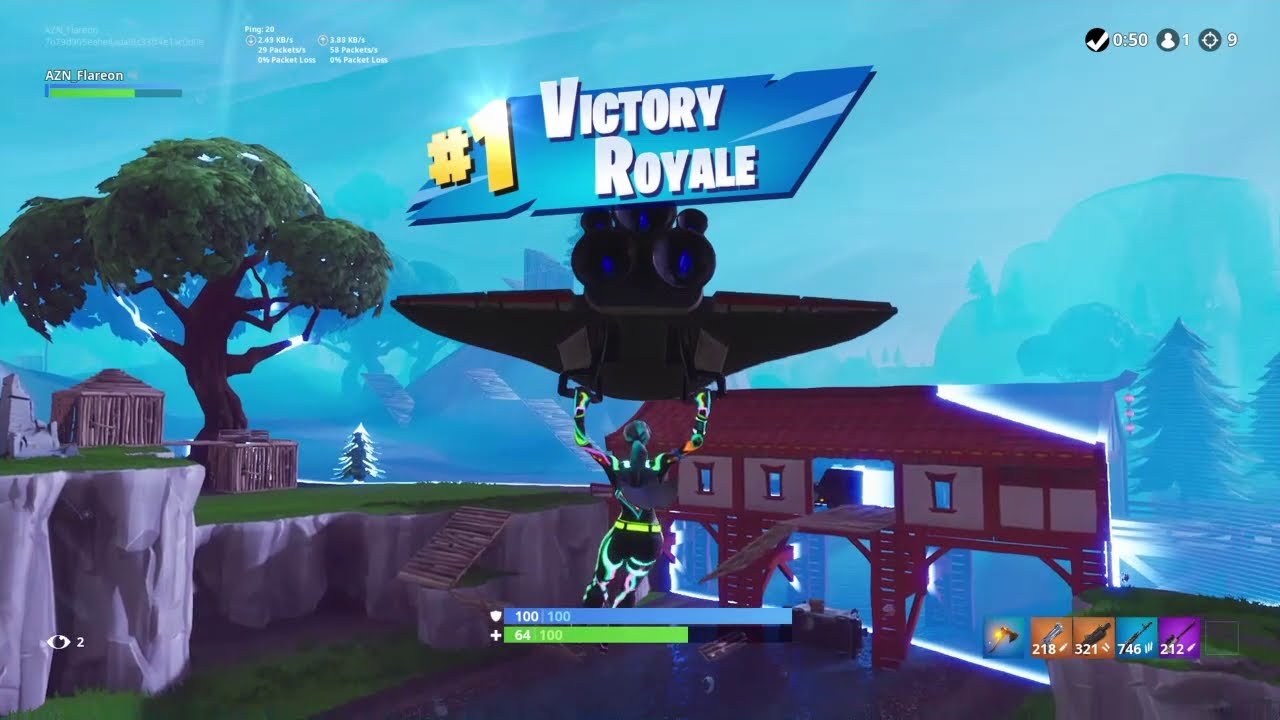This detailed image is a screenshot from a video game. Dominating the center is a woman character dressed in a colorful outfit, hanging from a small, black flying vehicle with two triangular-shaped wings and two blue lights resembling eyes. Above the aircraft, in bright blue and gold banner with sans serif, all-caps text, are the words "H1 Victory Royale," with "H1" in yellow and "Victory Royale" in white, boldly declaring the win. Behind and to the left of her, a tree stands on a land of grass atop a platform that looks like a small cliff, with stairs leading down to a lower level. Wooden crates lie next to the tree. In the background, a red house sits perched above the ground, illuminated with blue light. The upper part of the background features a vivid blue sky, contrasting with a bluish fog that obscures distant, indiscernible trees. Game statistics are visible in the corners of the image, further emphasizing the in-game setting.